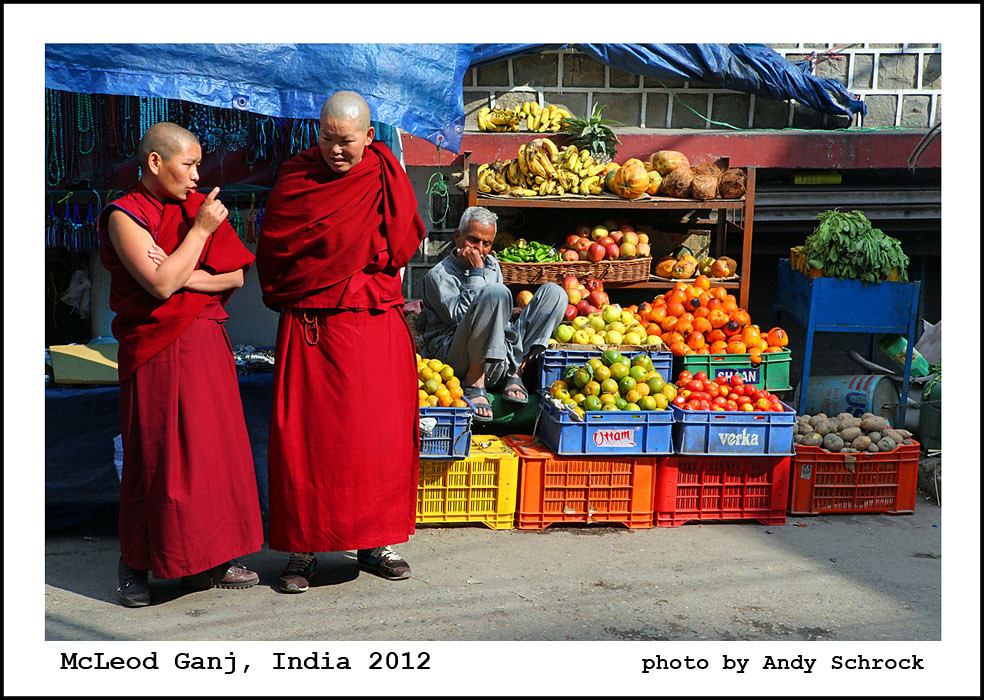The image depicts a vibrant scene at an open-air fruit and vegetable market in McLeod Ganj, India, dated 2012. The market setup consists of a wooden structure with shelves backed by a brick wall, and it is sheltered by a blue tarp. A man dressed entirely in gray, including his shirt, pants, and sandals, sits near the shelves of colorful produce. Surrounding him are an assortment of fruits and vegetables, including bananas, oranges, apples, tomatoes, spinach, and even potatoes, organized neatly in various colored crates and on the shelves behind him.

To the left side of the image, two monks with shaven heads, dressed in traditional red robes and brown shoes, are engaged in conversation. The scene is framed with a slim black border inside a thicker white border, adding a classic photographic presentation. At the bottom of the image, a caption reads: "McLeod Ganj, India, 2012. Photo by Andy Schrock." This highly detailed composition captures the bustling yet serene atmosphere of the market and the cultural essence of the locale.